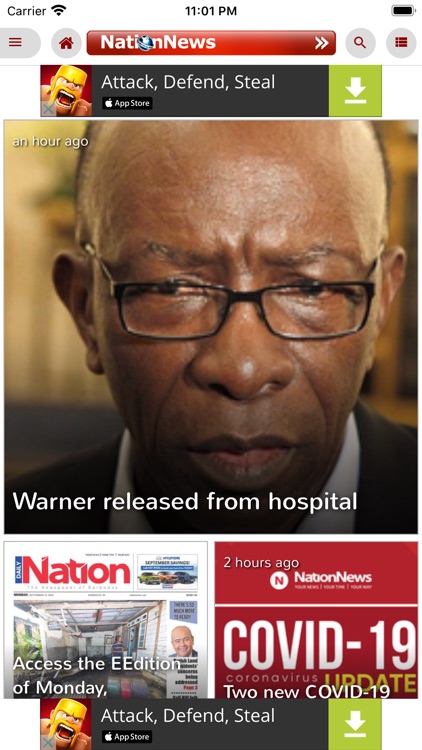At the top of the screen, the status bar shows "Carrier," a Wi-Fi symbol, and the time "11:01 PM" centered. On the right side of the status bar, a battery icon is visible. Below the status bar, a series of navigation and action buttons appear.

On the left side, three red lines are displayed against a dark gray background. Adjacent to this, there is a dark gray house icon, also in red.

To the right of this, there’s a red and maroon rectangle that contains "Nation News" alongside a circle symbol resembling the Earth in cyan blue and white. To the right of the Earth symbol are two white arrows pointing right. Encasing the rectangle is a gray circle with a red magnifying glass, and another gray circle with three bullets and three lines.

Beneath these controls, a banner for the game "Clash of Clans" depicts a character with a golden helmet and beard, yelling. Next to this character, a gray box with a teal 'X' inside displays the words "Attack, Defend, Steal" in white text. The background is black, and beneath it is a darker black rectangle displaying the Apple App Store logo—an apple with a bite taken out of it in white. To the right, a forest green square with a white down arrow and line symbolizes downloads.

Also visible is a news section featuring an African American individual. The top left corner of this section notes "an hour ago" in white, and the headline "Warner Released from Hospital" is presented in bold white text.

Lastly, the same "Clash of Clans" banner appears at the bottom of the screen.